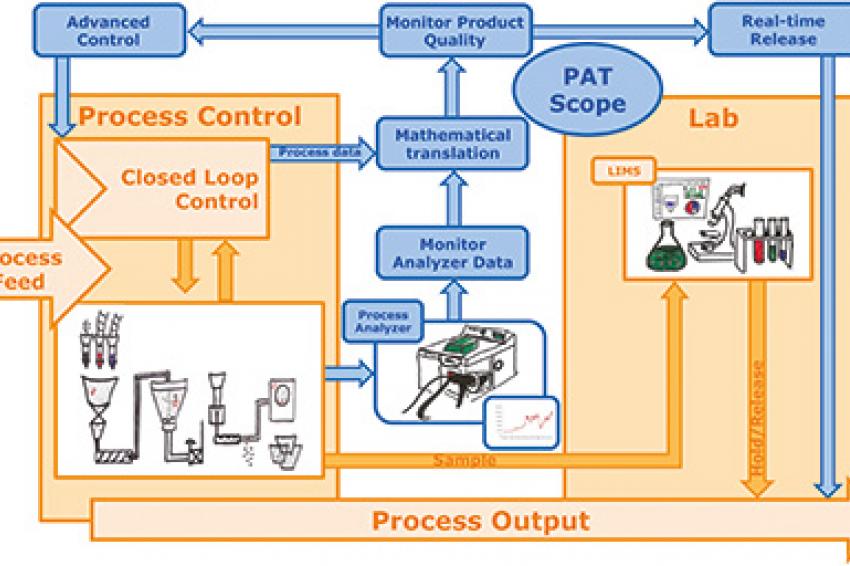The image depicts a detailed, science-related flowchart primarily in shades of blue, orange, and white. Starting from the top left, there is a blue box labeled "Advanced Control," which leads downwards through a series of arrows indicating a process. Directly under "Advanced Control," the flowchart transitions into a large orange box marked "Process Control," followed by "Closed Loop Control." The left side also features a graphical representation of scientific apparatus, including beakers leading into a contraption within a white square bordered by orange.

In the central section, from top to bottom, the flowchart details stages labeled "Monitor Product Quality," "Mathematical Translation," "Monitor Analyzer Data," and "Process Analyzer." Each of these stages includes corresponding diagrams to facilitate understanding. 

On the right-hand side, another prominent orange box is labeled "Lab," containing illustrations of scientific instruments such as a beaker with green liquid, a series of test tubes, and an animated microscope. At the top right, the label "Real-Time Release" is visible, with "Path Scope" positioned to its left. 

At the bottom of the flowchart, there is an overarching bar labeled "Process Output," encapsulating the final stage of this scientific procedure. The visual scheme and structure collectively emphasize the interconnectedness of control processes, quality monitoring, and lab analysis in real-time scientific applications.